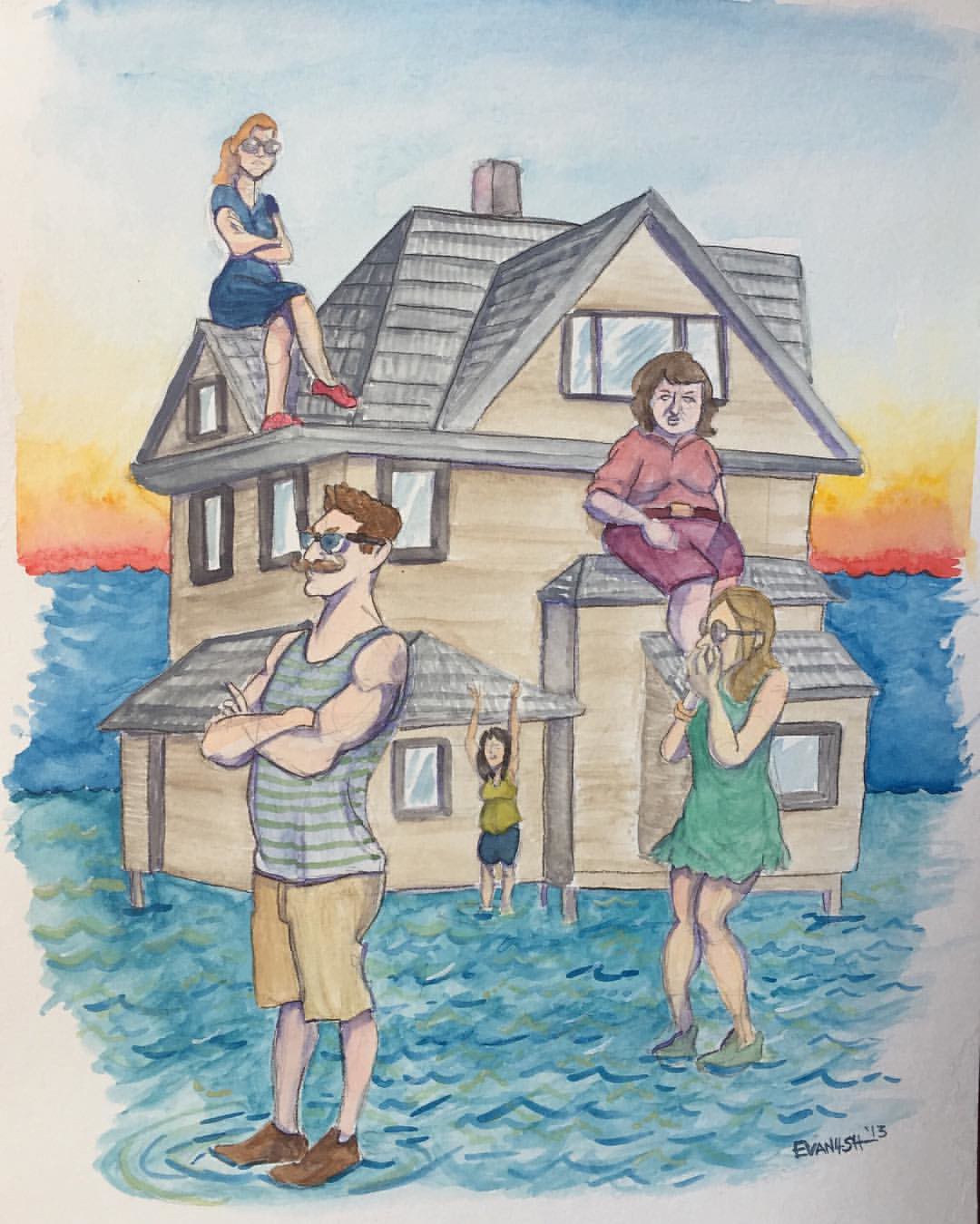This detailed artwork, likely a colored pencil drawing, features a brown two-story house with numerous windows, a dark gray roof, and a red chimney, all set against the backdrop of an ocean during a vibrant sunset with reds and yellows. The house appears to be atop wooden posts, surrounded by shallow, wavy water. Perched on a dormer of the roof is a woman with blonde hair, glasses, a blue dress, and red shoes, sitting cross-armed, her expression suggesting distress. On a lower section of the roof stands another woman in dark red pants, a lighter red shirt, and a belt, her brown hair flowing. Below her, a blonde woman also in glasses, dressed in a green dress and green shoes, covers her mouth with both hands as if gasping. Closer to the house, another woman in blue shorts and a pea-green shirt raises her arms. In the foreground, a man with brown hair and a mustache, wearing a gray and green striped tank top, khaki shorts, and brown shoes, stands with arms crossed, gazing to the left. The serene yet troubled scene is signed in the lower right corner, appearing as "Evan something SH13," and dated 2015.